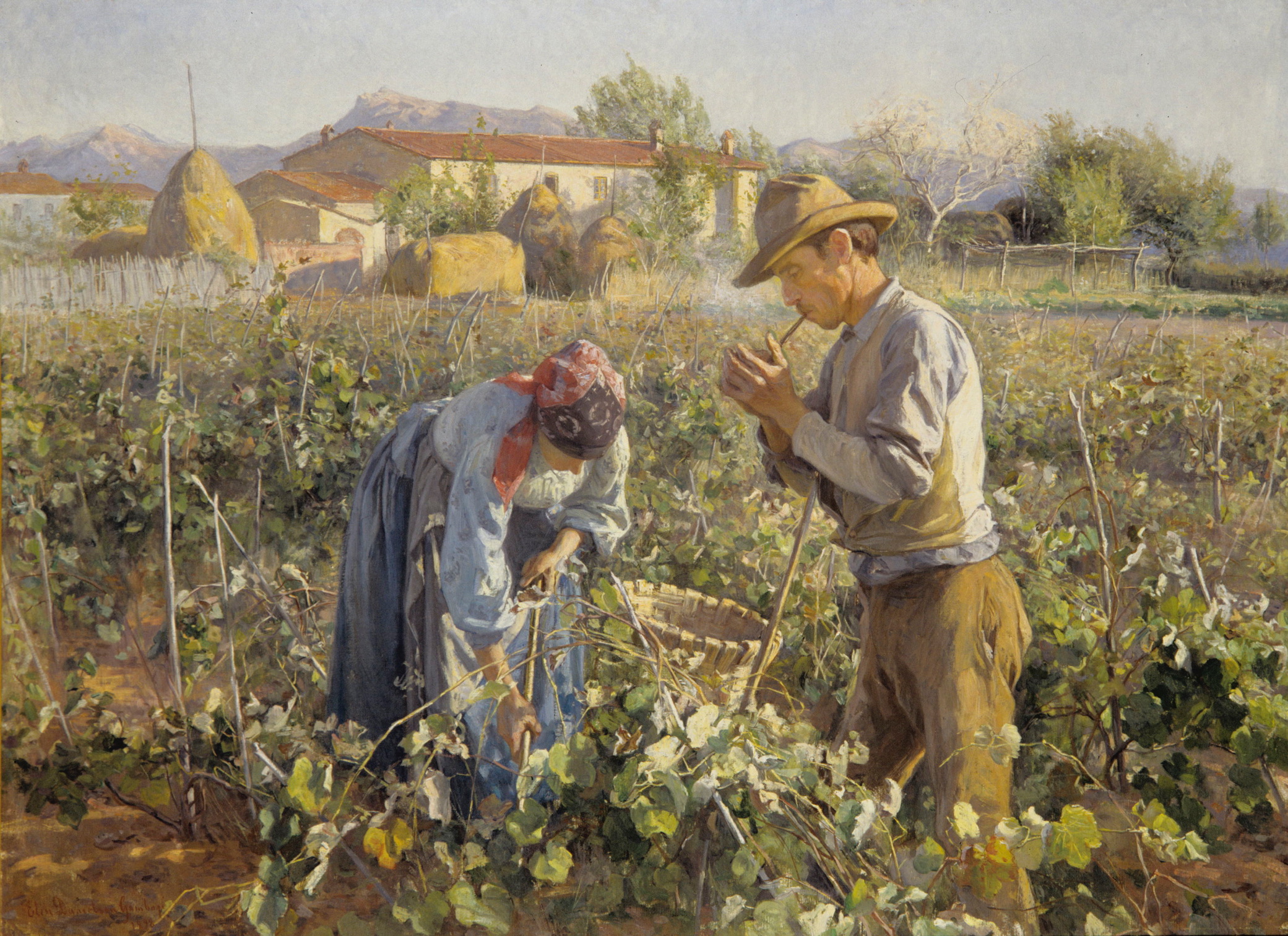The painting, done in a realistic style, depicts a man and a woman in a lush, green field. The woman, dressed in an old-fashioned blue skirt, blue top, and red bandana, is bent over, diligently gardening and plucking flowers or vegetables. Beside her is a grey basket, presumably for collecting her harvest. The man stands nearby, wearing a hat, blue shirt, and brown trousers, as he nonchalantly lights a cigarette. His actions contrast sharply with the woman’s hard work, creating a casual yet telling scene of everyday life. In the backdrop, the detailed landscape features a charming farmhouse with a red tiled roof and white walls, set amidst greenery with small huts, trees, and distant hills under a clear blue sky. Various gardening tools, such as a barrel and a bowl, are scattered between them, emphasizing their labor.